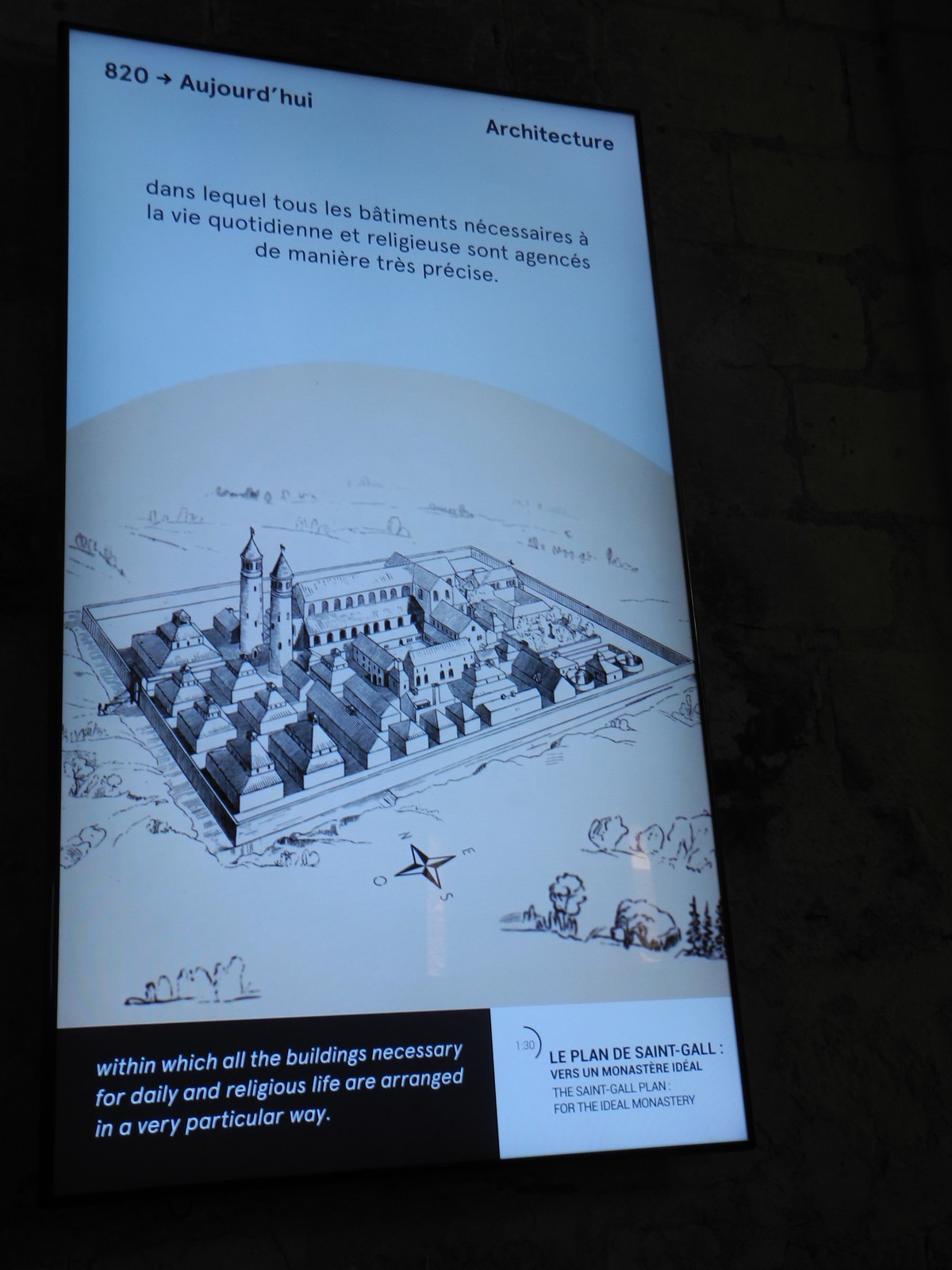The photograph captures a dark room with a warmly lit sign. The sign, set against either a dark brick wall or plain black background, seems to belong to a museum exhibit. It features a detailed drawing of an ancient city or castle, showcasing various buildings and towers necessary for daily and religious life, meticulously arranged within walls. The text on the sign is primarily in French, with some English translations. At the top of the sign, it reads "820, Architecture," followed by a French paragraph. The bottom of the sign includes an English notation: "within which all the buildings necessary for daily and religious life are arranged in a very particular way." This appears to refer to the "le plan de Saint-Gall," the Saint-Gall plan, which is known as the ideal monastery layout. The scene gives an almost grayscale impression with hints of black, white, gray, tan, and light blue, focusing on the historical and architectural significance of the depicted plan.